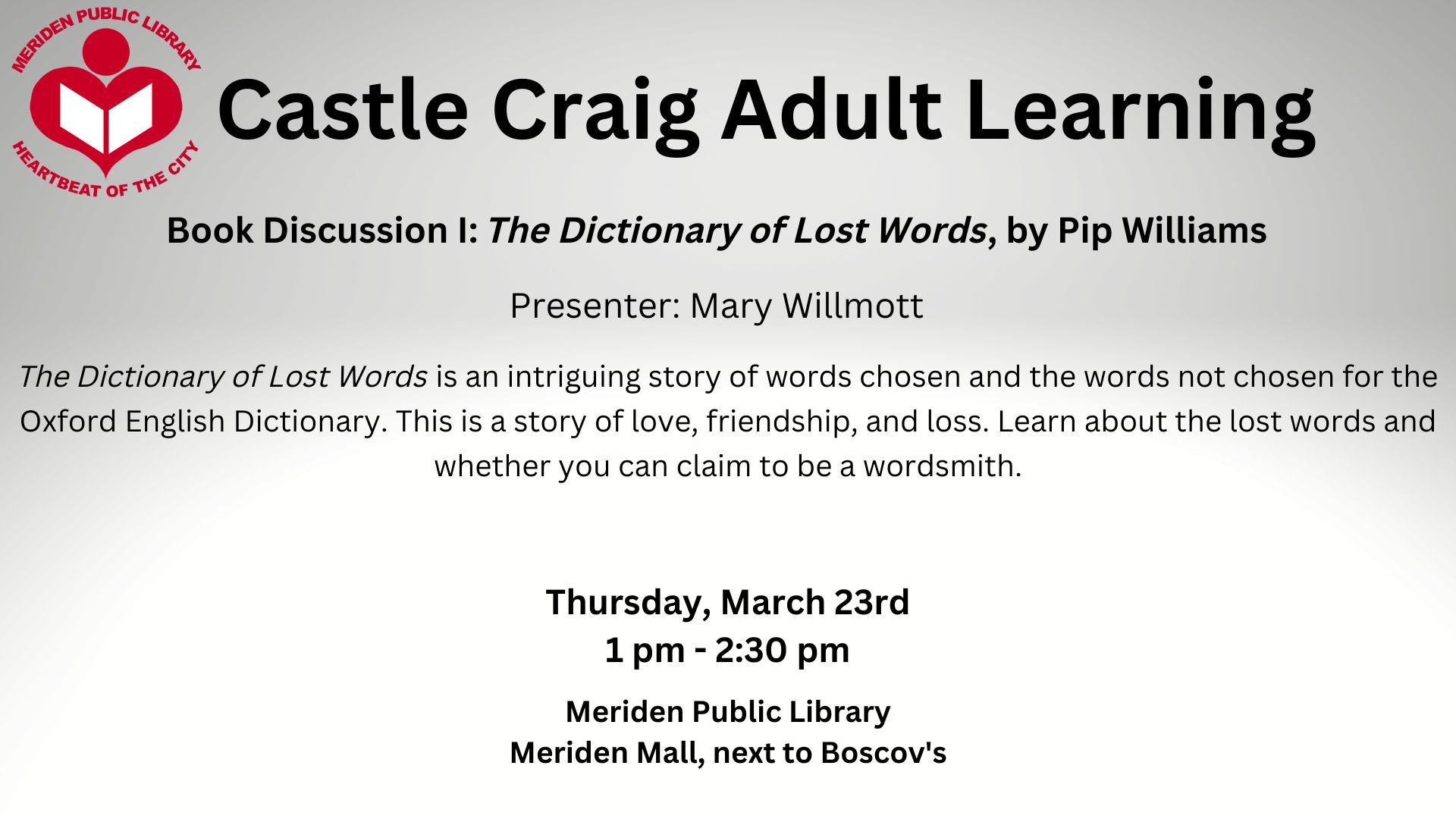The image is a horizontally rectangular print piece without a border. It features a gradient background that fades from gray at the top to white at the bottom. In the upper left corner, there is a red logo depicting a heart with a circle on top, resembling a head, and a white open book inside. Surrounding the logo, the text reads "Meriden Public Library" in a circular pattern at the top and "Heartbeat of the City" at the bottom. To the right of the logo, the text reads "Castle Craig Adult Learning." Below this, it announces "Book Discussion 1: The Dictionary of Lost Words by Pip Williams," presented by Mary Wilmot. This upcoming book discussion highlights "The Dictionary of Lost Words" as an intriguing story about the words chosen and not chosen for the Oxford English Dictionary, exploring themes of love, friendship, and loss. It invites participants to learn about the lost words and see if they can claim to be wordsmiths. The event is scheduled for Thursday, March 23rd, from 1:00 to 2:30 p.m. at the Meriden Public Library in the Meriden Mall, next to Boscov's.